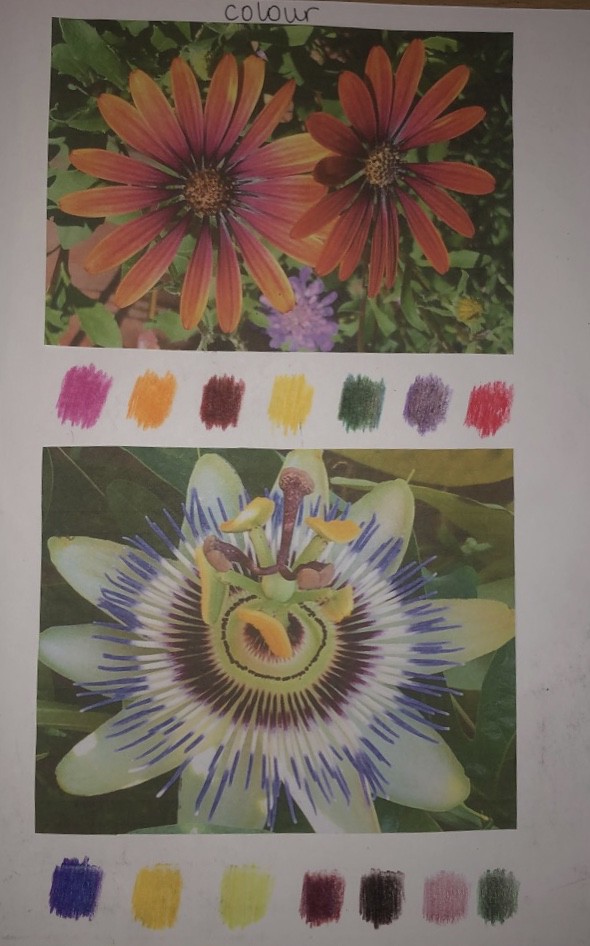The image features a striking collage of nature's vivid palette. The background is a pristine white, serving as a clean canvas for the color spectacle that unfolds.

On the top left, there is a gradient display beginning with soft pink hues, transitioning through vibrant orange, deep brown, and sunny yellow, then continuing to lush green, rich purple, and finally a bold red. This color sequence sets a warm, inviting tone for the entire image.

The very bottom left showcases a series of color swatches: blue, yellow, light green, brown, green, pink, green, and pink again. These swatches mirror the colors found in the images below, creating a harmonious blend throughout the composition.

The top image features two radiant red flowers, each with a striking yellow gradient. Their petals are vibrant and eye-catching, set against a lush background of green leaves that add a natural contrast.

The middle section darkens slightly, drawing attention to an orange-centered blossom surrounded by an array of green leaves. A solitary purple flower at the bottom adds a pleasing pop of complementary color to this section.

The final image on the bottom presents an extraordinary flower with a complex color pattern. Starting at the center, it bursts from green through fine brown stripes, to radiant white stripes, finally blending into soft bluish hues. The petals culminate in intensely green tips, and the leaves extending outward are lush, green, and vibrant, circling the flower and providing a vivid, dynamic frame.

Together, these images form a lush, colorful tapestry, highlighting the intricate beauty found in nature down to the finest details.